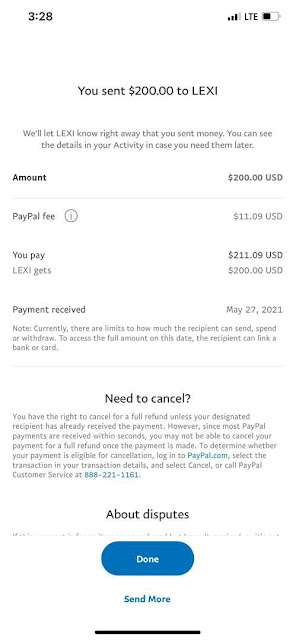Screenshot of a PayPal transaction confirmation screen showing that $200 has been sent to a recipient named Lexi. The total amount, including a PayPal fee, is $211.09. The screen advises notifying Lexi about the transfer and mentions that Lexi can check the details in her activity log. There is also a note indicating current limits on how much Lexi can send, spend, or withdraw until she links a bank account or card to access the full amount on a specified date. At the bottom, there are options to either click a "Done" button or a "Send More" button, both highlighted in blue. The screen clarifies the cancellation policy, stating that once a payment is received—usually within seconds—it may be hard to cancel for a full refund. To check eligibility for cancellation, one must log into PayPal and navigate to the transaction details or call customer service. The phone's battery appears to be about halfway charged.